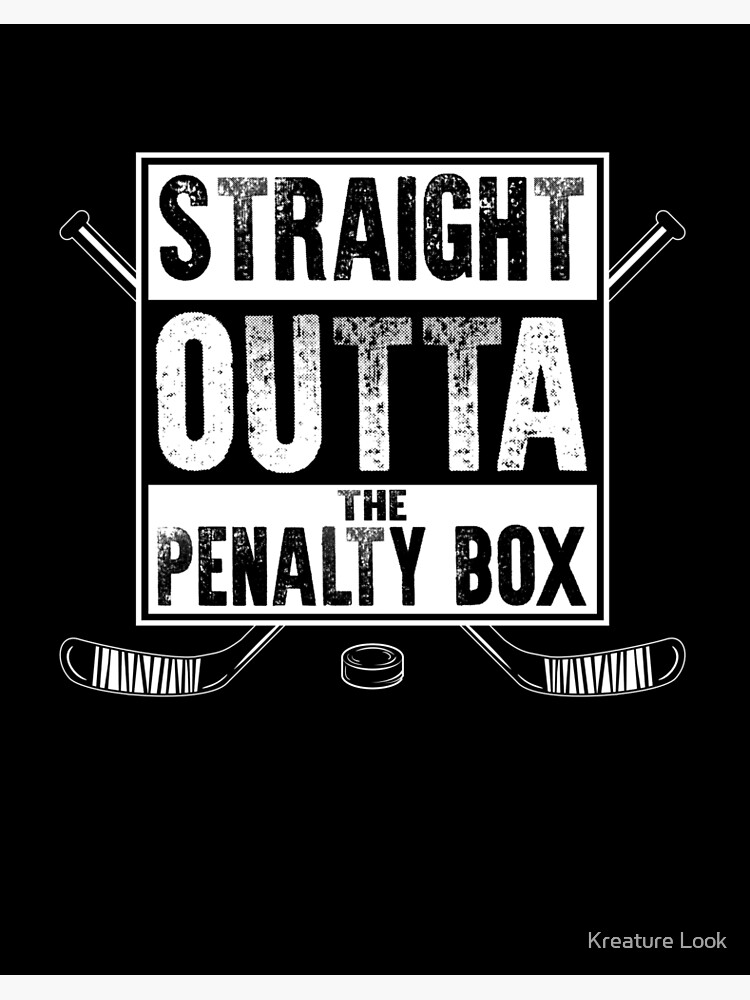The image features a digital poster set against a completely black background. Dominating the center is a prominent white-bordered square outlined again in black, which is divided into three horizontal sections. The top section features the word "STRAIGHT" in bold black letters on a white background. The middle section showcases "OUTTA" in striking white letters on a black background. The bottom section returns to a white background with the phrase "THE PENALTY BOX" printed in black. Overlaying this square are two crossed black hockey sticks, faintly adorned with white details, with their handles peeking out from behind the top section and their blades visible beneath the bottom section of the sign. Beneath this sign sits a solitary black hockey puck, outlined in white to enhance its visibility against the black background. In the bottom right corner, the text "Creature Look," distinctly styled as "K-R-E-A-T-U-R-E L-O-O-K," is displayed in grey. The entire composition is rendered in a monochromatic black-and-white scheme, emphasizing the stark contrasts and thematic elements of the design.